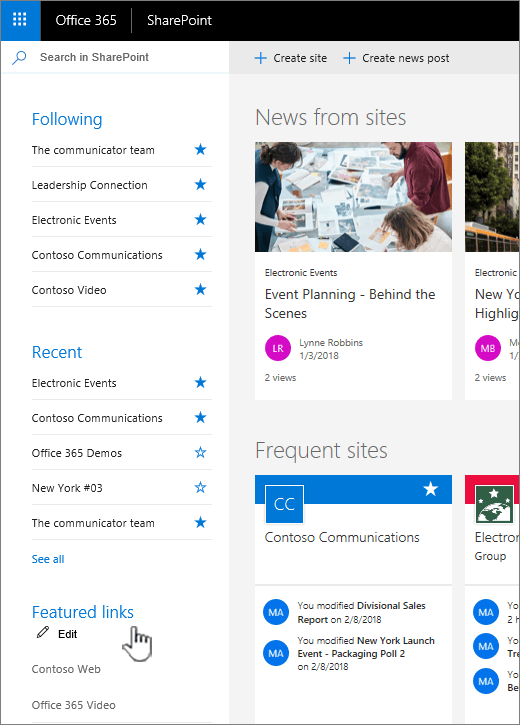This image showcases a detailed view of a SharePoint site within Office 365. At the top, a black navigation bar houses the label "SharePoint" and, to its far left, a blue square icon displaying nine white dots, which serves as a menu to access various options. 

On the left side of the interface, a vertical menu lists several links categorized as "Following," including "Communicator Team," "The Leadership Connection," "Electronic Events," "Contoso Communications," and "Contoso Video." These provide quick access to different sections and resources within the SharePoint site.

To the right, a white content area features a variety of clickable options such as "Recent Office 365 Demos," "Electronic Events," and "Featured Links," arranged in a vertical chronology as you scroll down the page. Additionally, there are several visual widgets that display images and other rich media, which are interactive elements.

Further to the right, there is a section titled "News from Sites," followed by another labeled "Frequent Sites." This part of the layout highlights commonly accessed or updated areas within the site. It prominently features "Contoso Communications," identifiable by the "CC" logo displayed above the link.

Towards the bottom of the page, a blue bar spans across with a star icon, symbolizing important information or a bookmark feature. Beneath this bar, there are two white circles with highlighted sentences indicating recent modifications, such as, "You modified divisional sales report," and "You modified New York launch event, Packaging Poll Two." These updates showcase changes and activities performed by users, providing a dynamic overview of the site's ongoing projects and content.